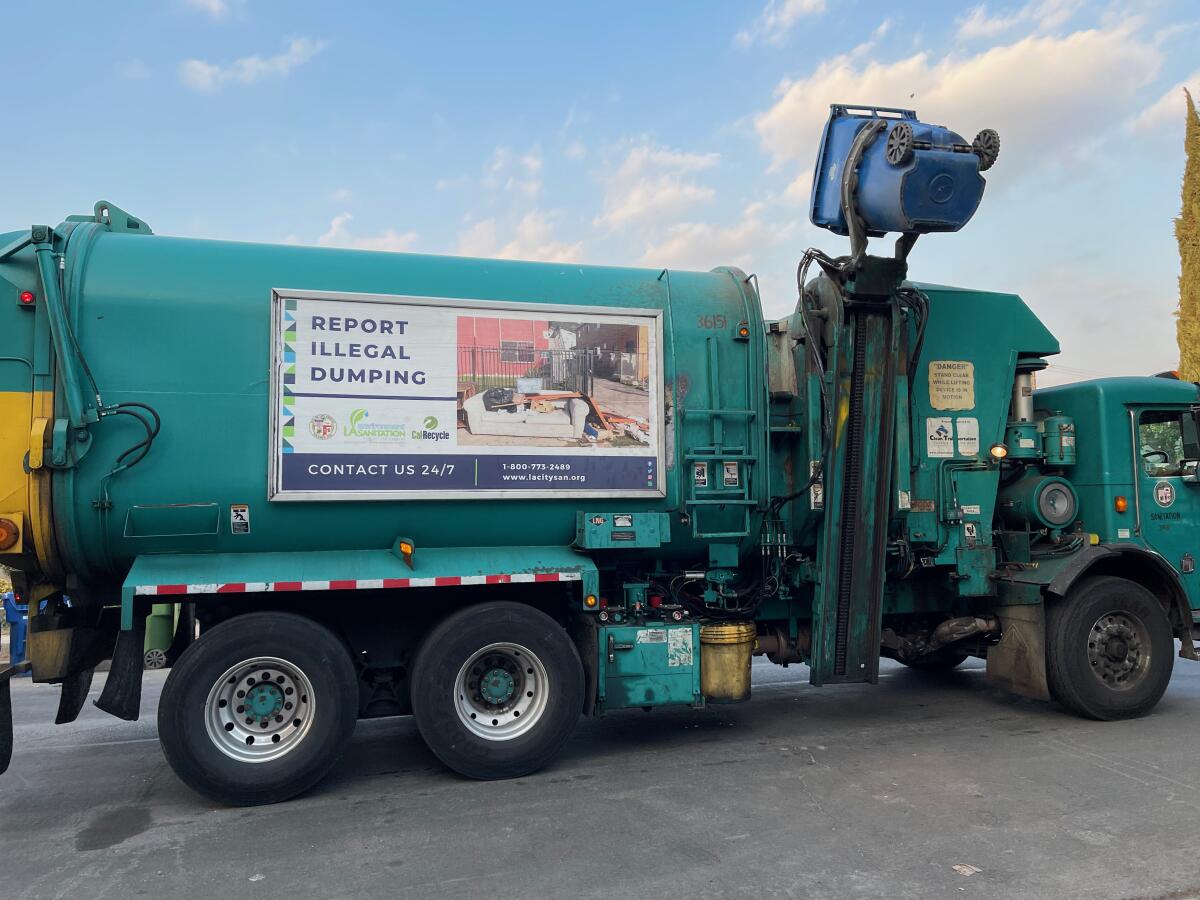This outdoor daytime photograph captures a large, teal green garbage truck with a mechanical arm elevated in the process of dumping a blue recycling bin into the top of the truck. The truck is parked on a cement surface under a clear blue sky. Prominently displayed on the side of the truck is a large sign that reads, "Report Illegal Dumping. Contact us 24-7," accompanied by an image of a discarded white couch surrounded by debris and trash. The back portion of the truck features yellow accents, and the overall appearance of the vehicle is notably dirty.